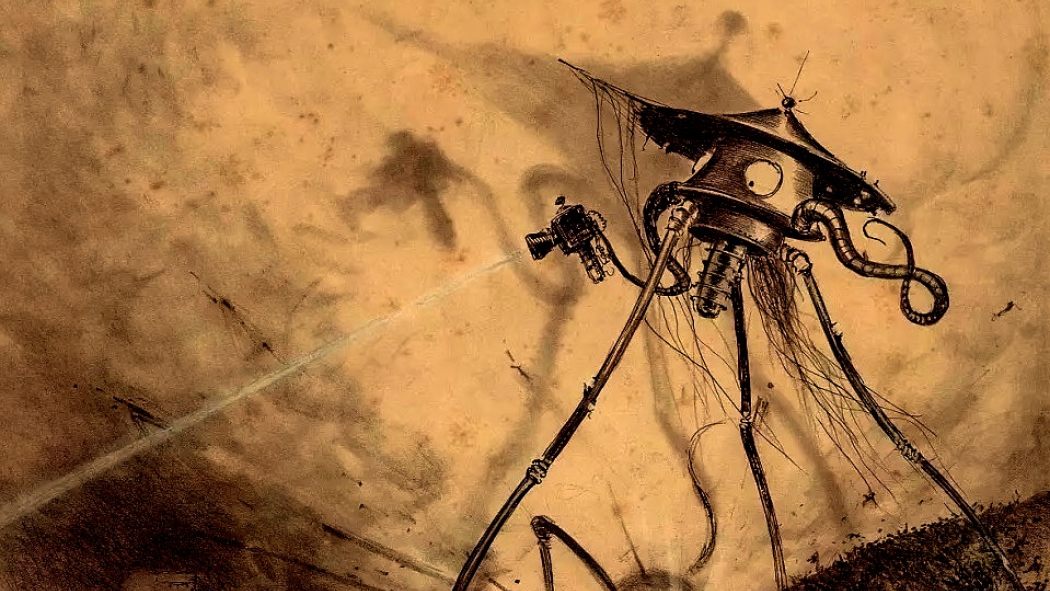The image is a detailed, artistic sketch, possibly handmade or illustrated, depicting a tin robot or alien-like figure. This character stands on three mechanical, tripod-like legs and has octopus-like tentacle arms. It sports what looks like a tin hat and possesses two distinctive eyes. One of its tentacles appears to be holding a ray gun, with a beam of light projecting forward. The background showcases an orangey-brown hue, adding to the vintage or rustic aesthetic. The figure’s shadow, including the ray gun, is visible against a rock face or similar terrain, emphasizing its presence. This imaginative and intricate design could be a creative piece meant for watering plants or a whimsical interpretation of an extraterrestrial with a weapon.